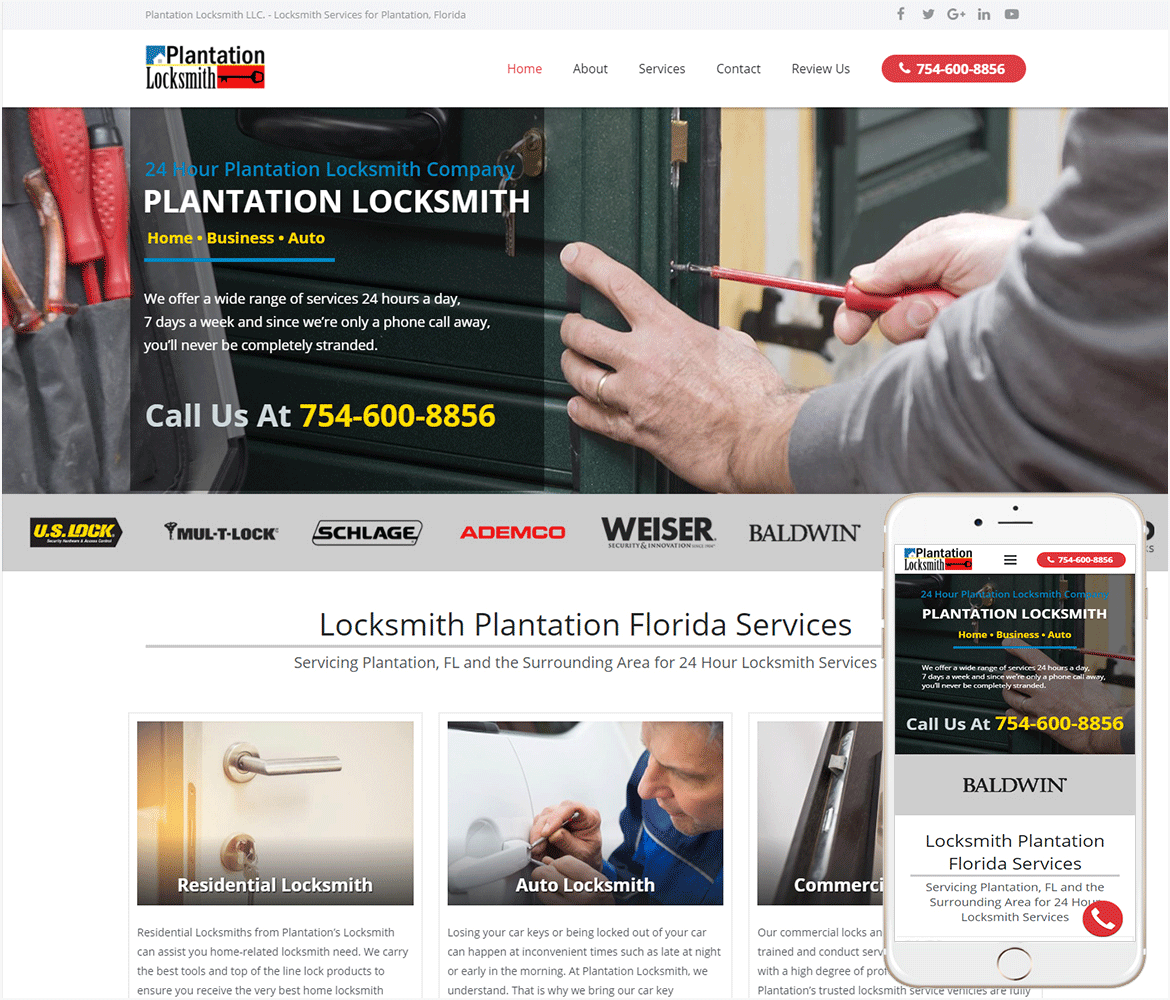A promotional graphic for Plantation Locksmith appears on a white background. At the top, there's a red oval with the text "Home" in red beside it. The image features a man fixing a door, holding a screw in his hand, under the banner "Plantation Locksmith Company." Surrounding the image is a detailed description of the locksmith services offered, affirming the availability of the company 24/7. A call-to-action message is included in yellow numbers, urging viewers to call 754-600-8856 for assistance. The bottom of the graphic displays several logos from renowned lock and security brands, including U.S. Lock, Multi-T Lock, Schalge, Ademco, Weiser, and Baldwin.